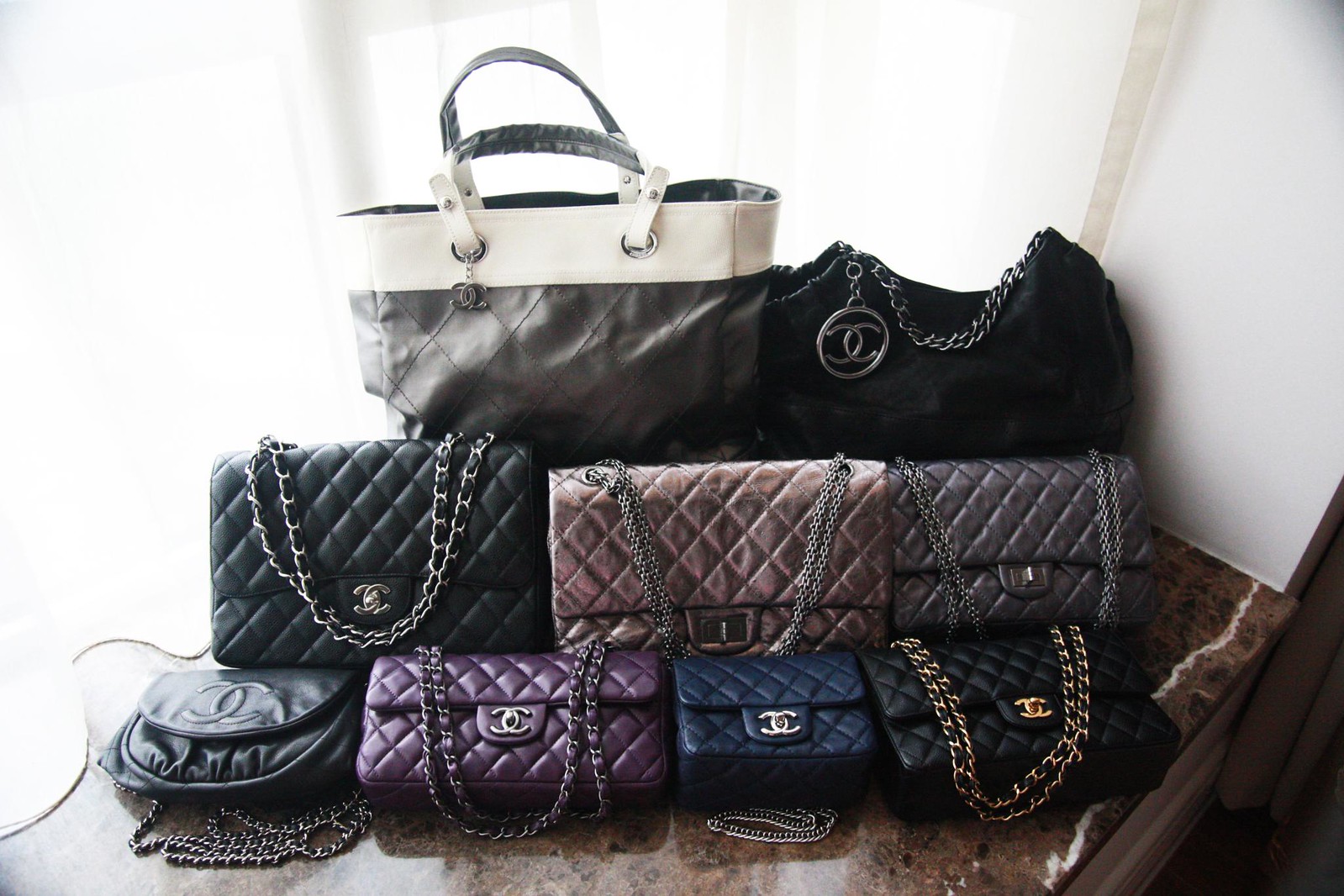This is a detailed colour photograph of ten leather-look handbags meticulously arranged in a pyramid shape on a glossy dark wooden table. The background features a large white wall with a window on the left, casting delicate shadows suggestive of a curtain. Dominating the apex of the pyramid is a white satchel-type bag with two short leather-look straps. Directly below are two slouch-style bags in charcoal gray. 

The second row from the bottom consists of three quilted handbags with silver chain handles: a black one with a silver chain handle on the left, a tan one with a silver chain handle in the center, and a gray one with a silver chain handle on the right. 

The bottom row showcases four smaller quilted handbags. They are distinguished by their chain straps, with a combination of black, blue, and gray bags alongside a notably smaller black quilted pouch. Additional details include a variety of chains in both gold and silver and occasional Chanel logos, particularly prominent on some of the front-row bags.